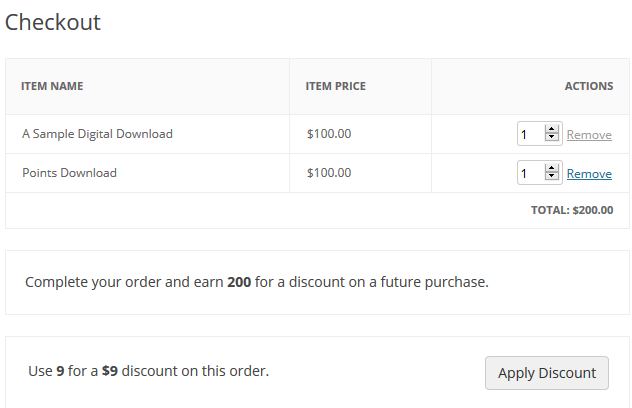This is a screenshot of an online shopping cart checkout screen, primarily featuring a clean, minimalistic design with a white background and gray text. At the top left corner, the word "Checkout" is prominently displayed. Below this heading, the checkout interface is organized into three distinct columns: one for item names, one for item prices, and one for actions.

In the "Item Name" column, there are two listed items: "Sample Digital Download" and "Points Download," each priced at $100. Under the "Actions" column, there are checkboxes to indicate the quantity, set to one for each item, and buttons to remove each item from the cart. The button for removing the "Sample Digital Download" is gray, while the button for removing the "Points Download" is blue.

At the bottom of the item list, the total purchase amount is displayed as $200. Beneath the shopping cart details, there is a message prompting users to "Complete your order and earn 200 for a discount on a future purchase." Below this, there is an option to "Use nine for a $9 discount on this order," accompanied by an "Apply Discount" button on the right-hand side.

The overall design of the screen is quite basic and sparse, suggesting that it might be part of a tutorial for a website or software application, rather than an actual checkout interface.